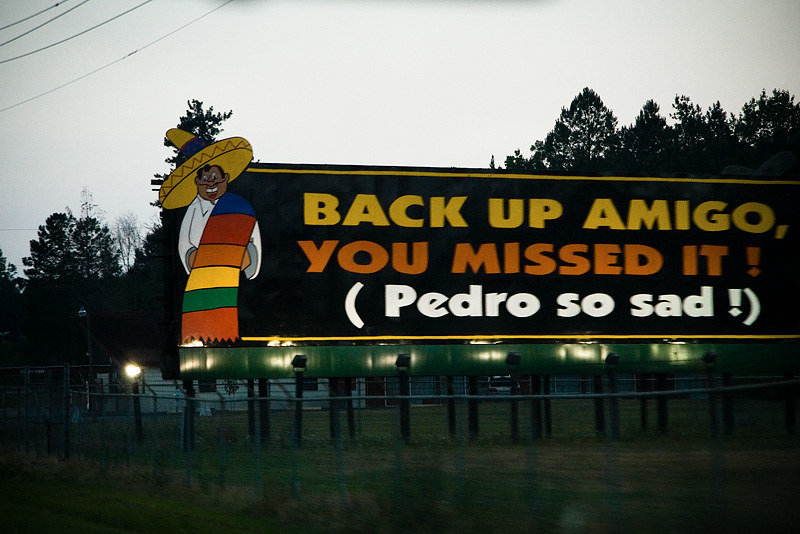The image features a prominently placed billboard sign against a backdrop of a white, cloudy sky. In the top left corner, electrical lines intersect the scene. Lush, green trees rise behind the billboard, while a metal fence stretches beneath it. The billboard is bordered in yellow and reads in bold, eye-catching colors: "BACK UP AMIGO," in yellow lettering, "YOU MISSED IT!" in red lettering, and "(PEDRO SO SAD!)" in white lettering. Towards the left side of the billboard is an illustration of Pedro, who has a darker skin tone. Pedro is depicted wearing a hat, a white shirt, and a rainbow-colored scarf over his shoulder. The billboard is illuminated by lights positioned at its bottom edge.